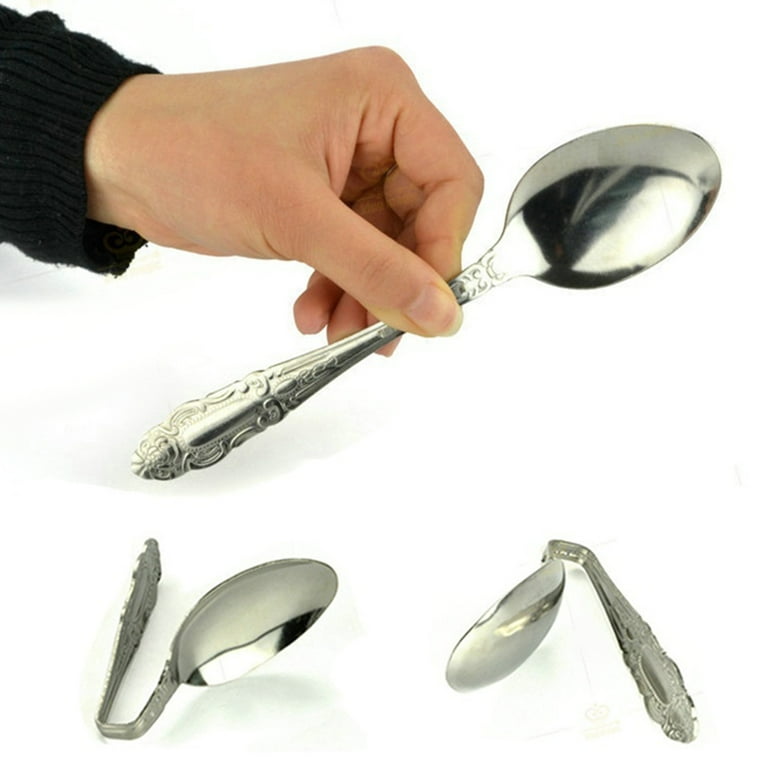The photograph is a vertically rectangular image with a pristine white background, showcasing three silver spoons staged in an indoor setting with artificial lighting. Dominating the top left of the image, a Caucasian woman's hand, distinguished by a long thumbnail, emerges from a dark navy blue long-sleeved top to hold the handle of a straight silver spoon with a decorative, engraved bottom. Directly below and to the left and right of this central spoon, two additional silver spoons are positioned, both noticeably bent and warped in different angles, revealing their intricate handles. The colors throughout the image include tones of white, silver, and dark navy blue, with subtle shades of gray and black from reflections on the metal.